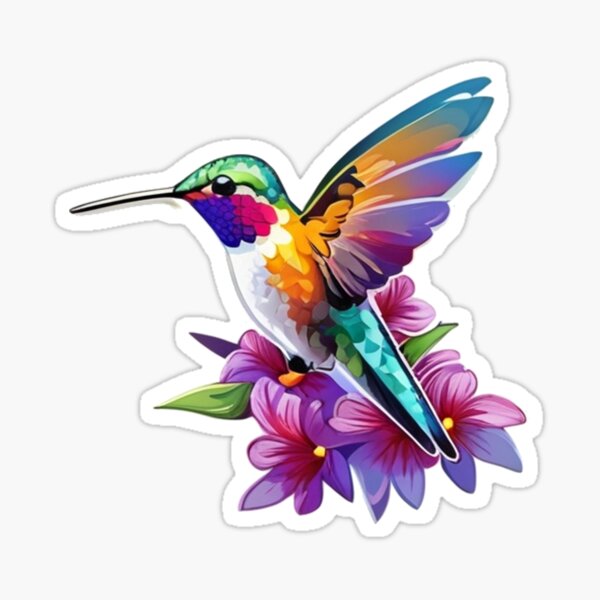This image features a vibrant, highly stylized sticker of a hummingbird against a white background. The hummingbird is depicted facing to the left with its wings extended up behind it, showcasing a stunning array of colors including green on the head and backside, a blue patch under its throat, and yellow, orange, and black on its wings with hints of purple and red. Its elongated, slender beak and distinctive eye, a prominent black with a reflective spot, add to its realistic portrayal. Surrounding the hummingbird are purple, pinkish-blue flowers with yellow centers and accompanying green leaves. The intricate details and rich color palette give the sticker a rainbow-like appearance, highlighting its artistic and possibly commercial purpose, such as an advertisement for purchase on platforms like Etsy or Amazon.